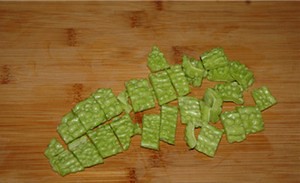The image depicts a light tan wooden floor, clean and free of any visible dirt, serving as the backdrop. Scattered on the floor are approximately 25 pieces of cut-up celery. The celery pieces, exhibiting a fresh, green appearance with slight moisture, seem to have been recently washed and diced, leaving the wooden surface somewhat damp. The pieces vary slightly in size and shape, with most appearing as flat, rectangular fragments. There are no cutting utensils or any other objects present, focusing the attention entirely on the neatly arranged, green vegetable pieces lying on the smooth wooden texture.